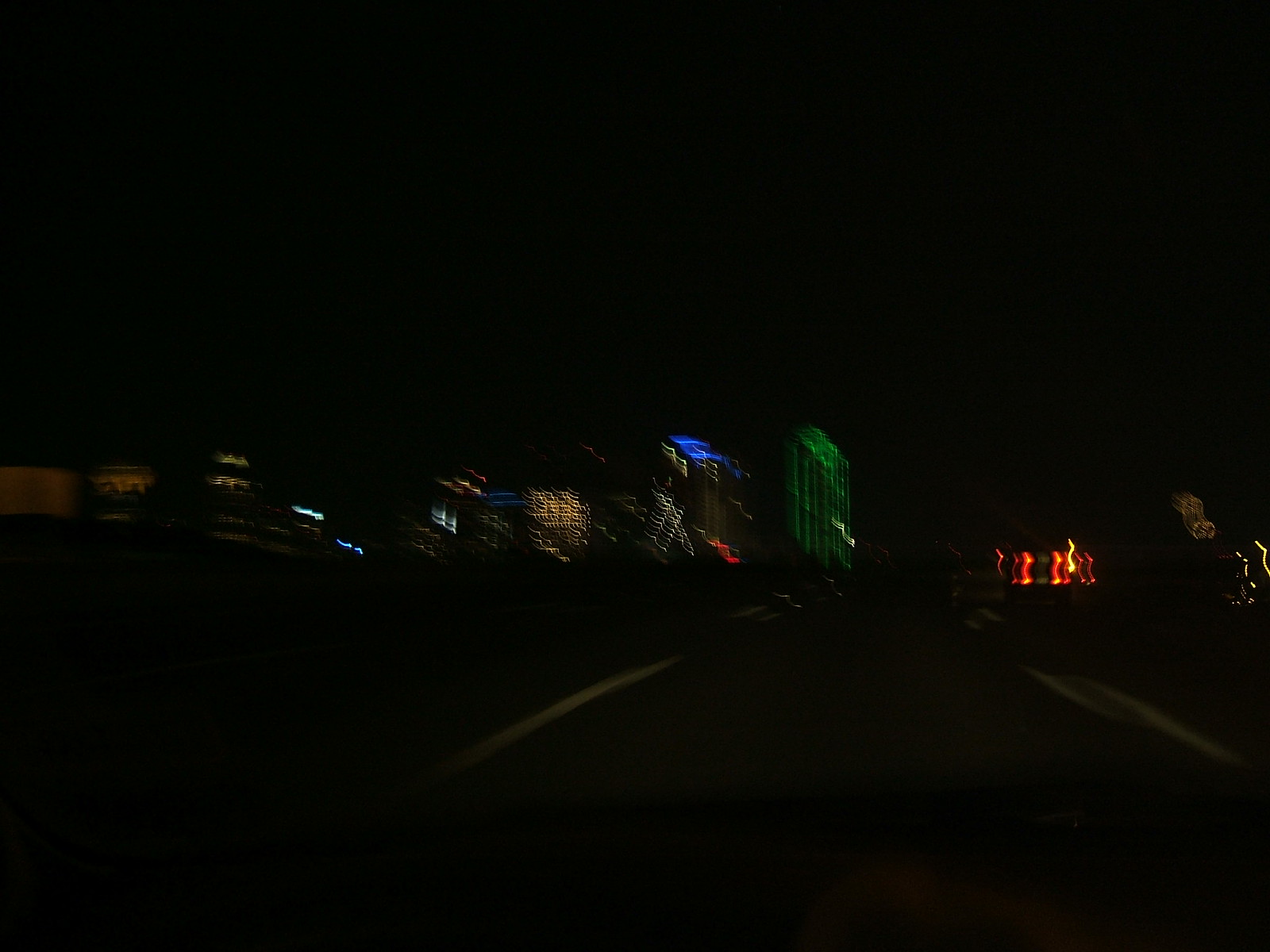This is a nighttime photograph capturing a blurry city street scene. The image is predominantly dark, with the top and bottom sections almost entirely black. At the center, a multi-lane road with white lines stretches out, leading towards the city. To the right, vibrant buildings display significant color variations: a sequence of bright lights in red, yellow, orange, and green draws attention. Specifically, there are yellow buildings, a green-lit facade, blue lights crowning another building, and an overall mixture of lights creating an X shape in the center. The fourth building stands out with vivid green lighting, while the last building features fiery orange illumination. Despite the overall blurriness, the scene effectively captures a bustling urban nightlife, illuminated by a spectrum of colorful lights against a dark backdrop.